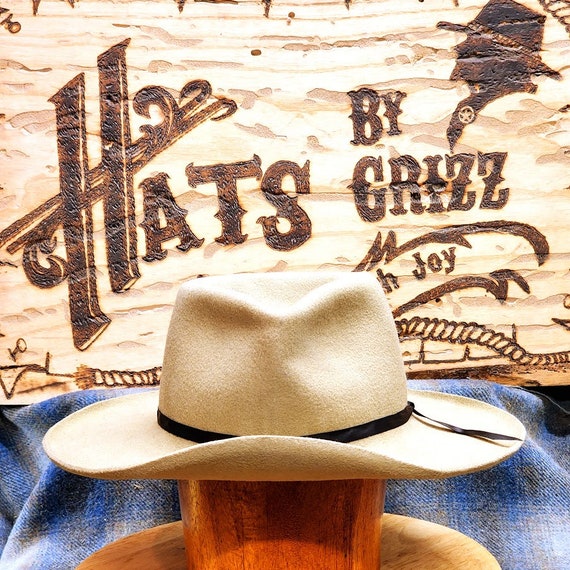The photograph captures a cream-colored Panama hat adorned with a black ribbon, elegantly placed atop a brown wooden log. Adjacent to the log lies a blue cloth, adding a splash of color to the scene. Behind the hat, there is a cream-colored board featuring dark brown text that reads "Hats by Chris Joy." In the top right corner of the board, a logo depicts a silhouette of a man wearing a hat, facing left. The composition suggests a promotional image, possibly taken in a brightly lit shop, showcasing the finely crafted hat by the creator.